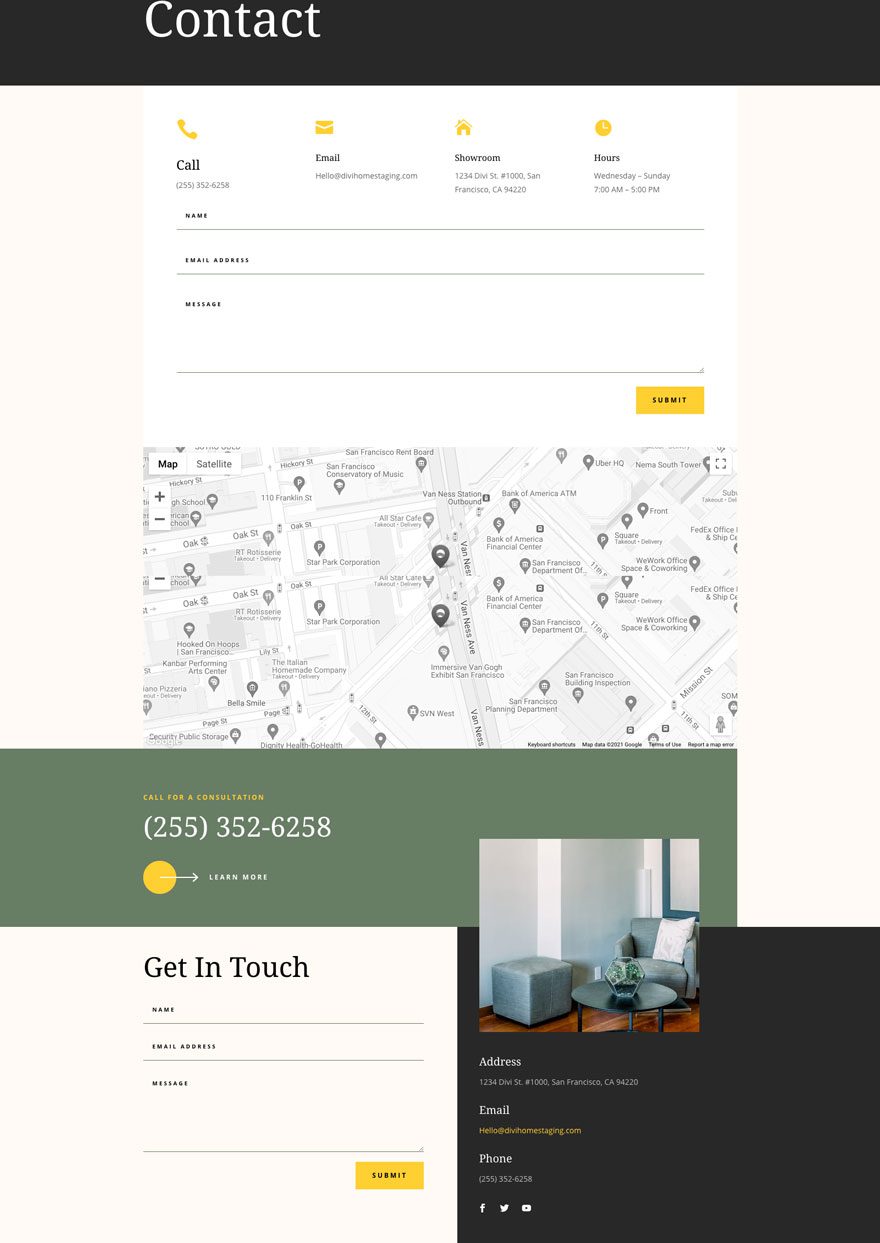**Contact Section of Interior Designer's Website**

The top banner of the contact section features a sleek black background with the word "Contact" displayed prominently in white lettering. Below this banner, the main content area begins with a clean white section that provides essential contact information. This includes:

- **Call:** The phone number listed for contact.
- **Email:** The specified email address.
- **Showroom:** The physical address of the showroom.
- **Hours:** The operating hours and days for visiting the showroom.

Further down, there is a user-friendly form with multiple input fields for visitors to enter their details and send a message. A "Submit" button is prominently displayed for easy form submission.

Adjacent to this form, a detailed gray map highlights the exact locations of the interior design firm's offices or showrooms. Beneath the map, a gray bar contains a call-to-action: "Call for a consultation" followed by the phone number 255-352-6258.

Below this, there is a yellow circle with a white arrow pointing to the right, next to the text "Learn More," acting as a clickable link for additional information. Following this, the section reads "Get in touch," with spaces to enter one's name, email address, and a message. There is also a yellow "Submit" button for sending inquiries.

To the right of these input areas, an image displays a beautifully decorated corner of a living room, showcasing the interior designer's work. This part of the section also reiterates the firm's address, email, and phone number for easy reference.